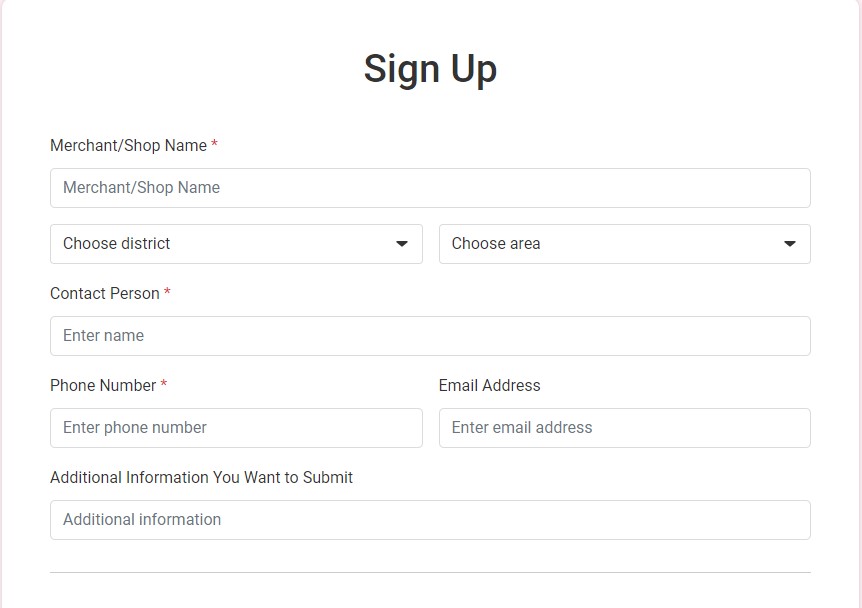The image is a detailed screenshot of a website's sign-up page designed for merchants or shop owners to register for a service. The page features a clean white background with various input fields and instructions. At the top center of the image, the prominent black text reads "Sign Up."

Immediately below, in slightly smaller black text, it is labeled "Merchant/Shop Name." A white dialog box outlined in gray, displaying the placeholder text "Merchant/Shop Name" in gray, indicates where users should enter the name of their business. 

Below this section, two drop-down boxes are presented side by side. The box on the left has black text that reads "Choose District," and the box on the right reads "Choose Area," both accompanied by black downward arrows, suggesting they are drop-down menus for selecting geographical locations.

Further down the page, in the center, there's a field labeled "Contact Person" with a gray placeholder indicating to "Enter Name." Underneath this, the left side of the page features a dialog box for "Phone Number," with the gray text prompting "Enter Phone Number." To its right, there is another dialog box labeled "Email Address," with the gray text "Enter Email Address" as the placeholder.

At the very bottom of the page, there is an additional input box for users to provide more details. It is labeled "Additional Information You Want to Submit" in black text, with the gray placeholder "Additional Information" inside the dialog box.

The layout is designed to guide users through the registration process step by step, ensuring that all necessary information is captured efficiently.